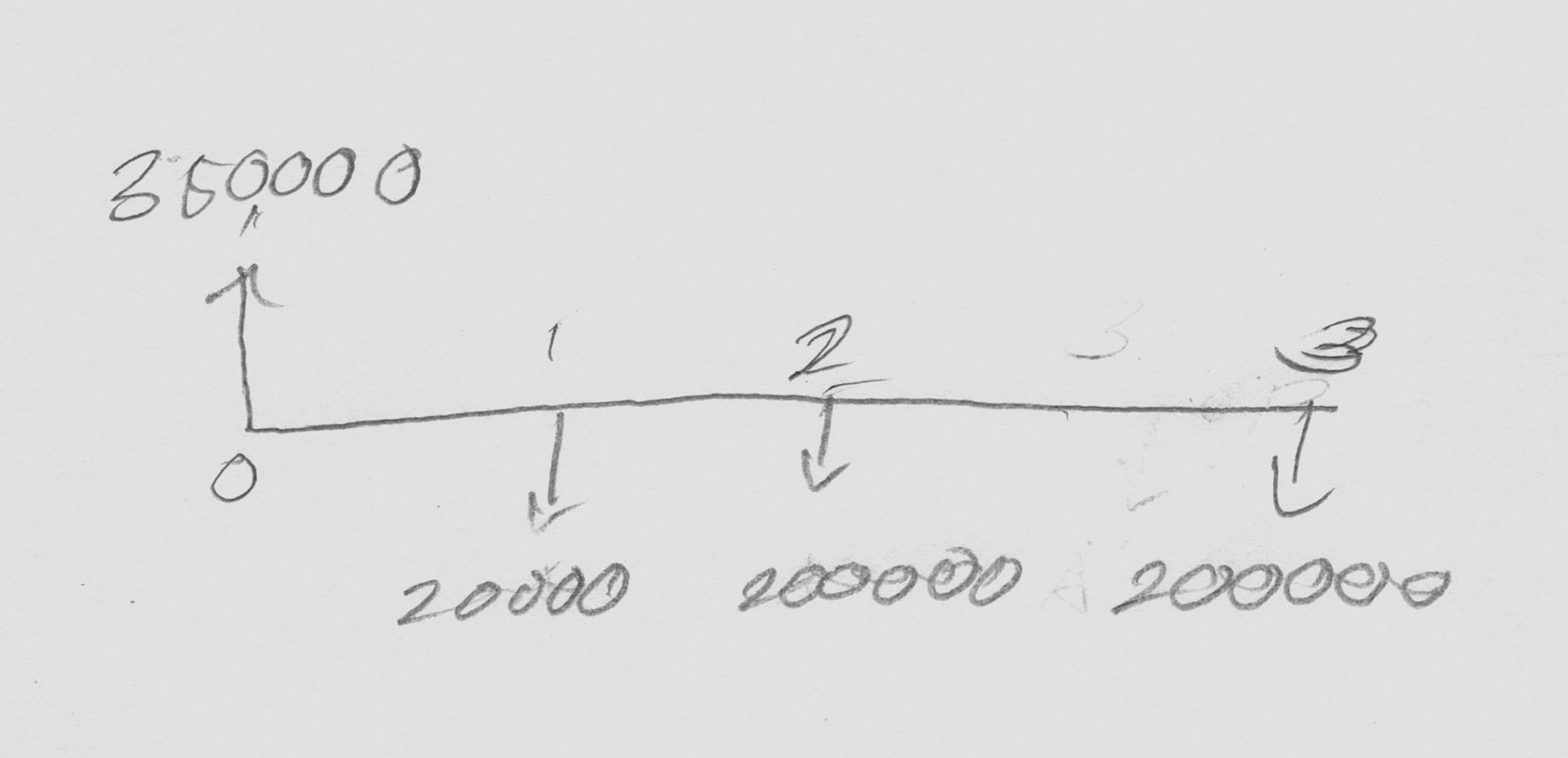A landscape-oriented piece of paper features a diagram sketched roughly in gray pencil. In the upper left corner, the number "350,000" is prominently displayed. Directly beneath this number, an arrow points upward before descending vertically and making a sharp right-hand turn, extending almost to the far right side of the page. Along this horizontal path are equally spaced numbers: "1," "2," and "3." The "3" is positioned at the far right edge, the "2" is in the middle, and the "1" is halfway between the "2" and the initial vertical arrow.

Below each of these numbers, small downward arrows lead to additional numerical values: "20,000" is situated below the "1," "200,000" beneath the "2," and another "200,000" under the "3." At the turning angle of the initial vertical arrow, near the left of the page, the notation "A0" is marked just below this angle.